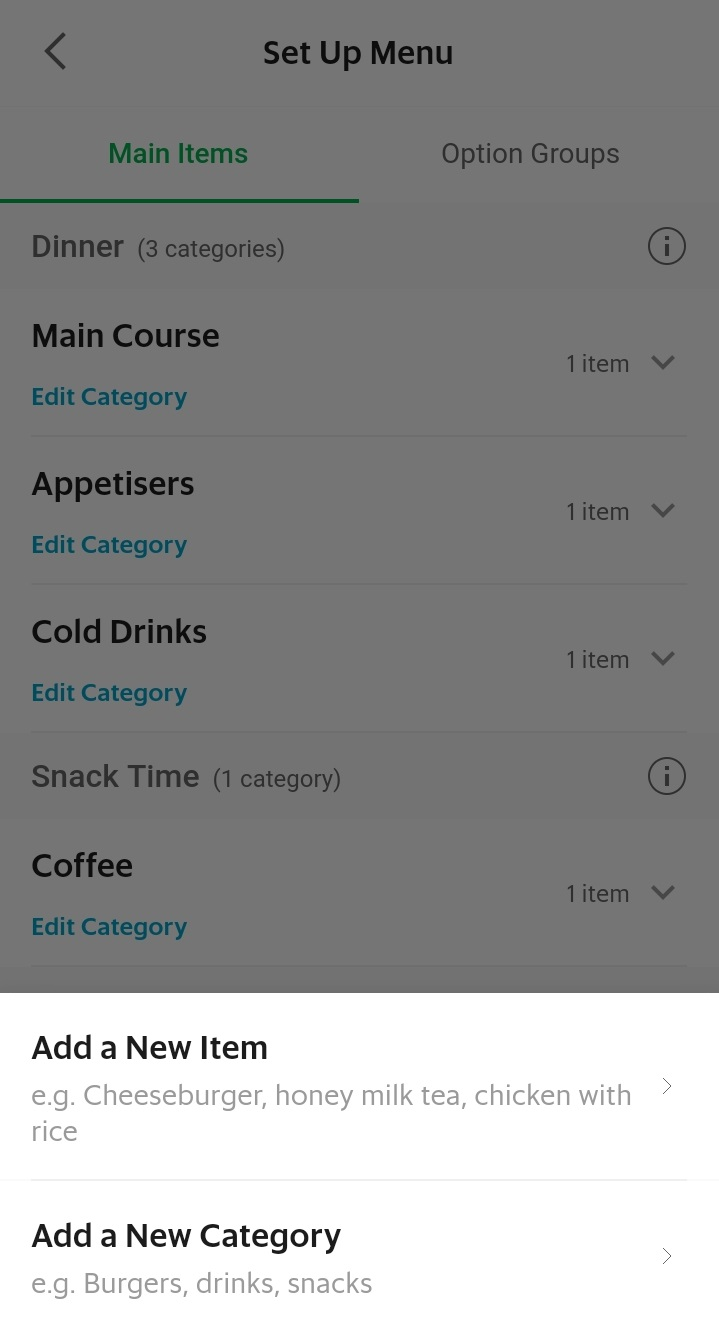The image depicts a dark, out-of-focus, smartphone screen showcasing a menu setup interface. The screen displays various colors to indicate different sections: grey signifies option groups, black is for the setup menu, green highlights the main items, and blue with white covers detailed options.

The menu is organized into distinct categories, beginning with "Main Course" which allows for editing and currently lists one item. Following this is the "Appetizers" category, also editable with one listed item. Moving down, there is a section for "Cold Drinks," marked in blue with editable details turning white upon selection. The "Snacks" category and a "Coffee" section follow the same format, each editable with one listed item.

Towards the bottom of the screen, greyed-out text prompts the user to "add a new item," offering examples like a cheeseburger or honey milk tea, and "add a new category," with suggestions such as burgers, drinks, and snacks. The lower portion seems to be more illuminated and possibly contains the main navigation menu, hinted by its white color contrasting the dark background.